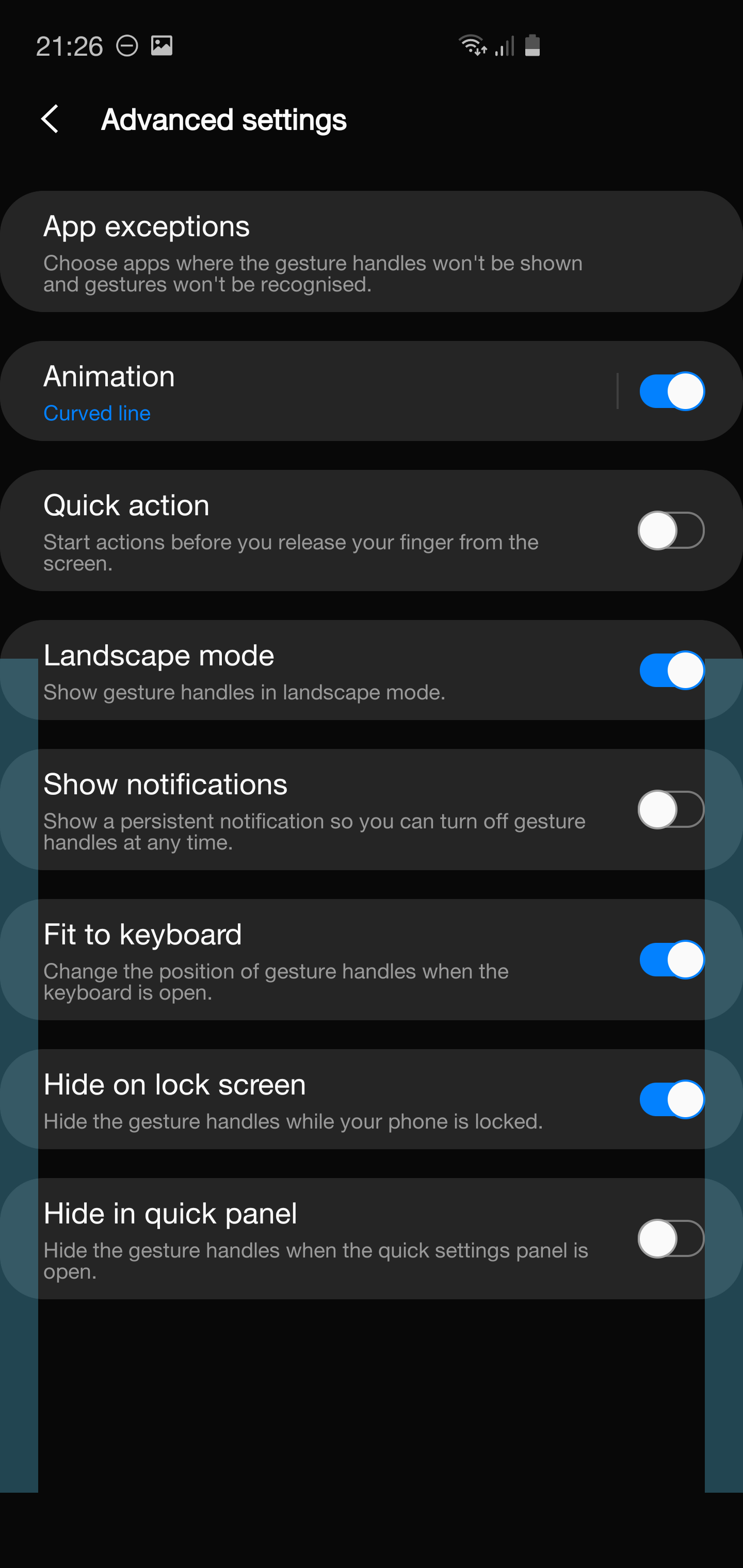A detailed screenshot of an app's "Advanced Settings" section reveals various customizable options for gesture controls:

1. At the top left, "Advanced Settings" is prominently displayed.
   
2. The first section is titled "App Exceptions," allowing users to choose specific apps where gesture handles will not be shown and gestures won't be recognized.
   
3. Below this, the "Animation" section includes an "Animation" option with a curved line, which is toggled on, as indicated on the right side of the screen.
   
4. Next is the "Quick Action" section, featuring the option to "Start actions before you release your finger from the screen." This feature is currently toggled off.

5. In "Landscape Mode," there is an option to "Show gesture handles and escape in landscape mode," which is toggled on.
   
6. The "Show Notifications" section includes "Show persistent notifications, so you can turn off gesture handles at any time," currently toggled off.

7. For keyboard settings, there's an option to "Change the position of gesture handles when the keyboard is open," which is toggled on.
   
8. The "Hide on Lock Screen" option allows users to hide the gesture handles while the phone is locked, and this is toggled on.
   
9. Lastly, the "Hide in Quick Panel" option, which hides the gesture handles when the quick settings panel is open, is toggled off.